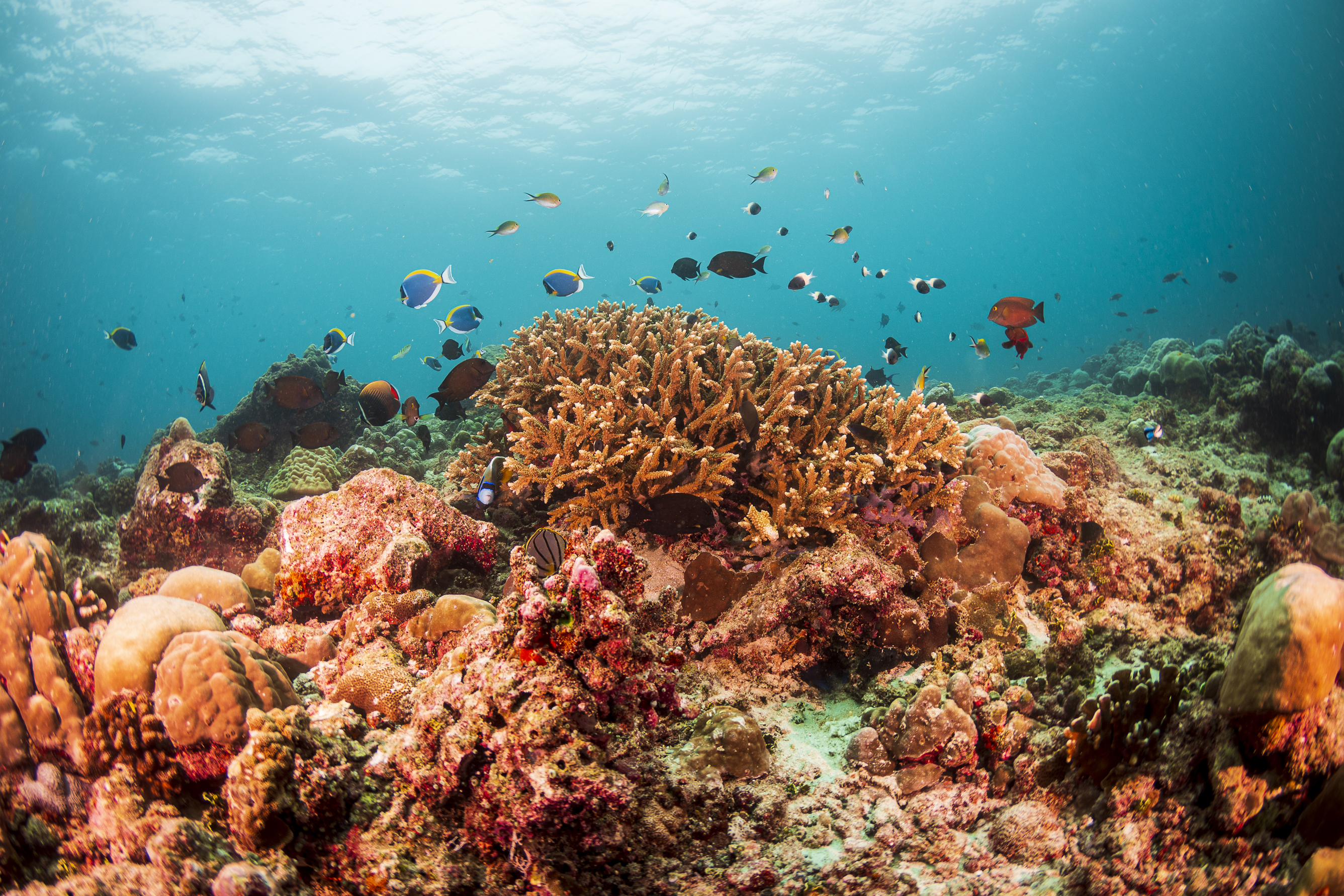This captivating underwater scene showcases a vibrant coral landscape teeming with life. The foreground is dominated by a diverse array of corals and sea anemones in vivid hues of reds, pinks, yellow ochres, oranges, and greens. These corals form the foundation of this richly textured marine environment. Above the coral, a variety of tropical fish swim, exhibiting a stunning spectrum of colors and patterns. Notably, a bright blue fish with a yellow marking on its back, a black fish, a rusty-colored fish, and several black-and-white fish stand out among the schools. Some fish are so distant that their features blur into the background, but their presence forms an intricate dance around the corals. The crystal clear blue water extends upwards, where the light from the sun filters through, casting a luminous glow from the center-left and creating a mesmerizing texture at the surface. The interplay of light, colors, and marine life creates an enchanting underwater tableau that is both dynamic and serene.